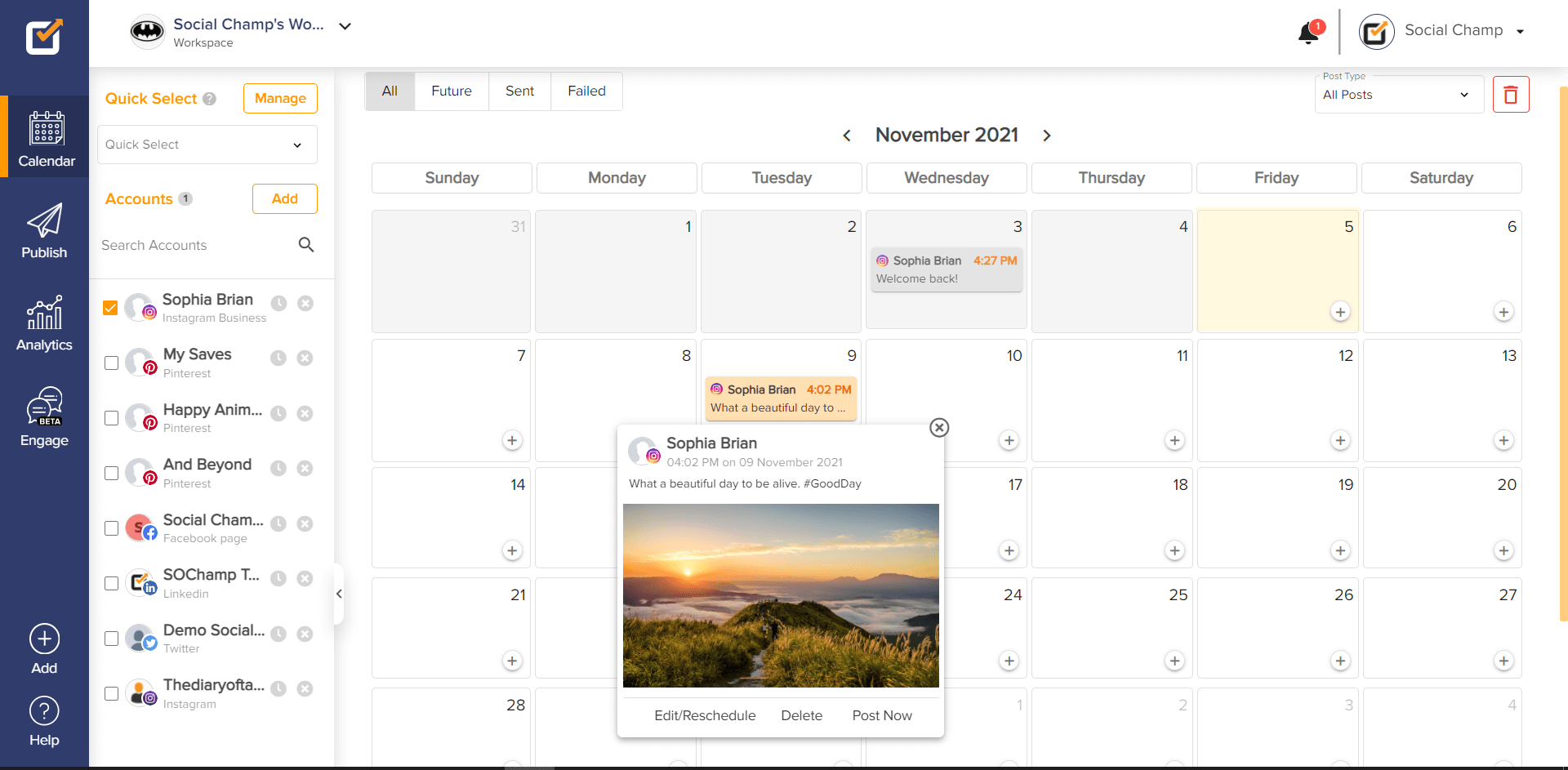The image is a detailed screenshot from Social Champs Workspace, showcasing various functional panes and a calendar interface. 

On the far left, there is a narrow, blue pane that displays four vertically stacked icons: a calendar icon labeled "Calendar," a paper airplane labeled "Publish," a bar and line graph labeled "Analytics," and two talk bubbles labeled "Engage." Below these icons, there are an "Add" button and a "Help" section.

Adjacent to this is a wider pane with a white background featuring a "Quick Select" in orange, a "Manage" button also in orange, an "Accounts" section, and an orange "Add" button. At the top, there's a "Search Accounts" bar. The pane lists several names, one of which is "Sophia Bryan," associated with an Instagram business account. Next to Sophia Bryan's silhouette avatar is an orange checkmark.

The main section of the webpage is a calendar titled "November 2021," spanning from Sunday to Saturday. On November 9th, there is an orange event bubble reading "Sophia Bryan, 4:02 p.m., What a beautiful day," linking to a detailed pop-up. The pop-up provides further details: "Sophia Bryan, what a beautiful day to be alive #goodday," posted at 4:02 p.m. on November 9, 2021, along with a panoramic landscape image. At the bottom of this picture, there are options to "Edit," "Reschedule," "Delete," or "Post Now."

Additionally, on November 3rd, there is a gray event bubble from Sophia Bryan at 4:27 p.m. with the text "Welcome back."